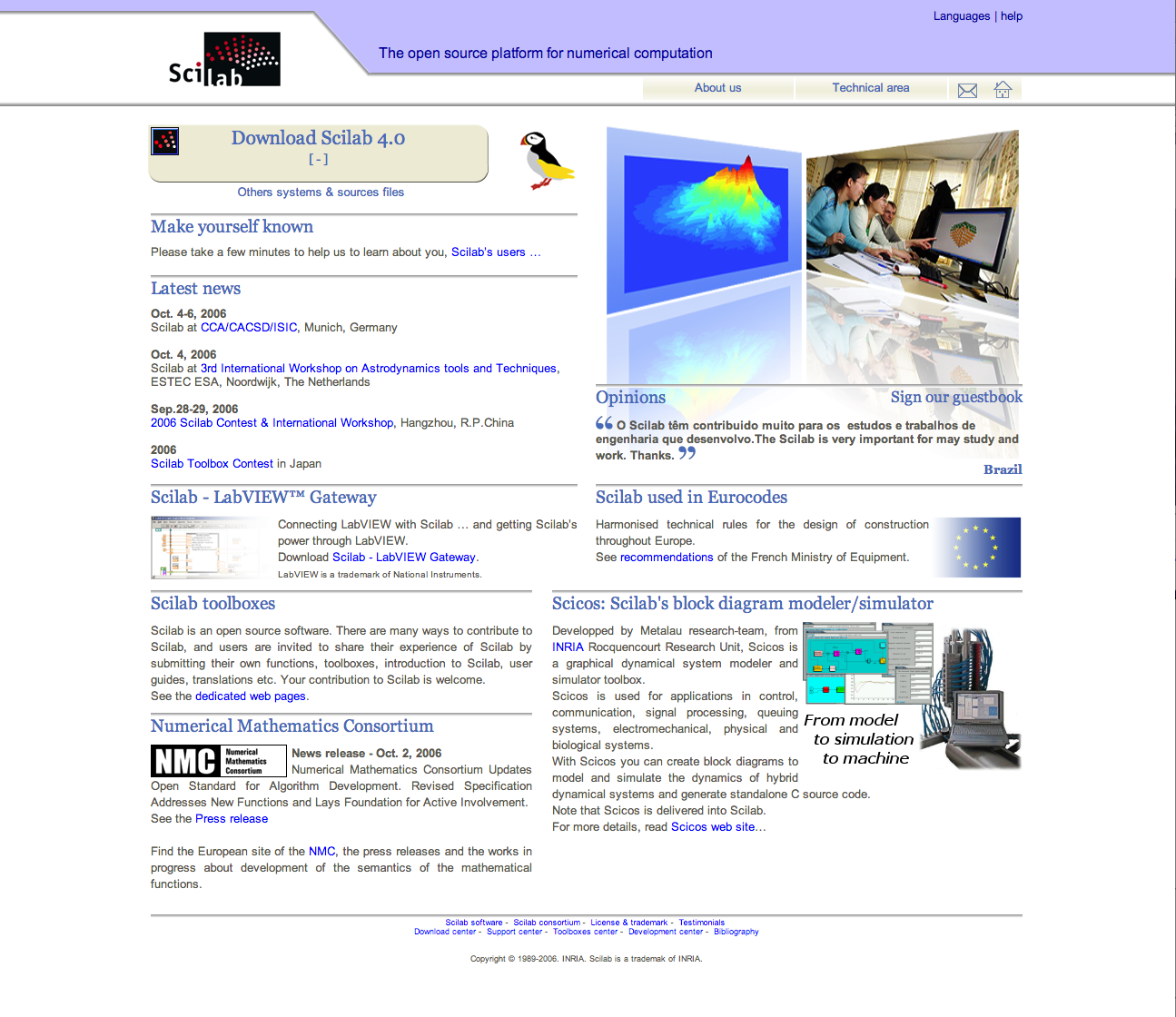Under the category "Website," there is a prominent gray navigation bar across the top displaying the tagline, "The Open Source Platform for Numerical Computation." This bar includes links for "Language" and "Help."

Beneath and slightly to the left of the gray bar is a black square featuring a pattern of red and white dots forming a half-arc. This square contains the word "Scilab," with "Sci" in black letters and "lab" in white letters. Below this square, text reads "Download Scilab 4.0," accompanied by a clickable link. Standing next to this section is a small puffin figure, facing to the left.

To the right of the puffin, there are two adjacent windows. The first window has a gray border with a vibrant blue interior, displaying an image resembling a volcano. The image transitions from blue at the base to orange, and then red, suggesting it might be a thermal map. Directly next to this window, the second window presents a scene of a few people gathered around a monitor. One individual is pointing at the screen while others sit around a table, all engaged and focused on the same display.